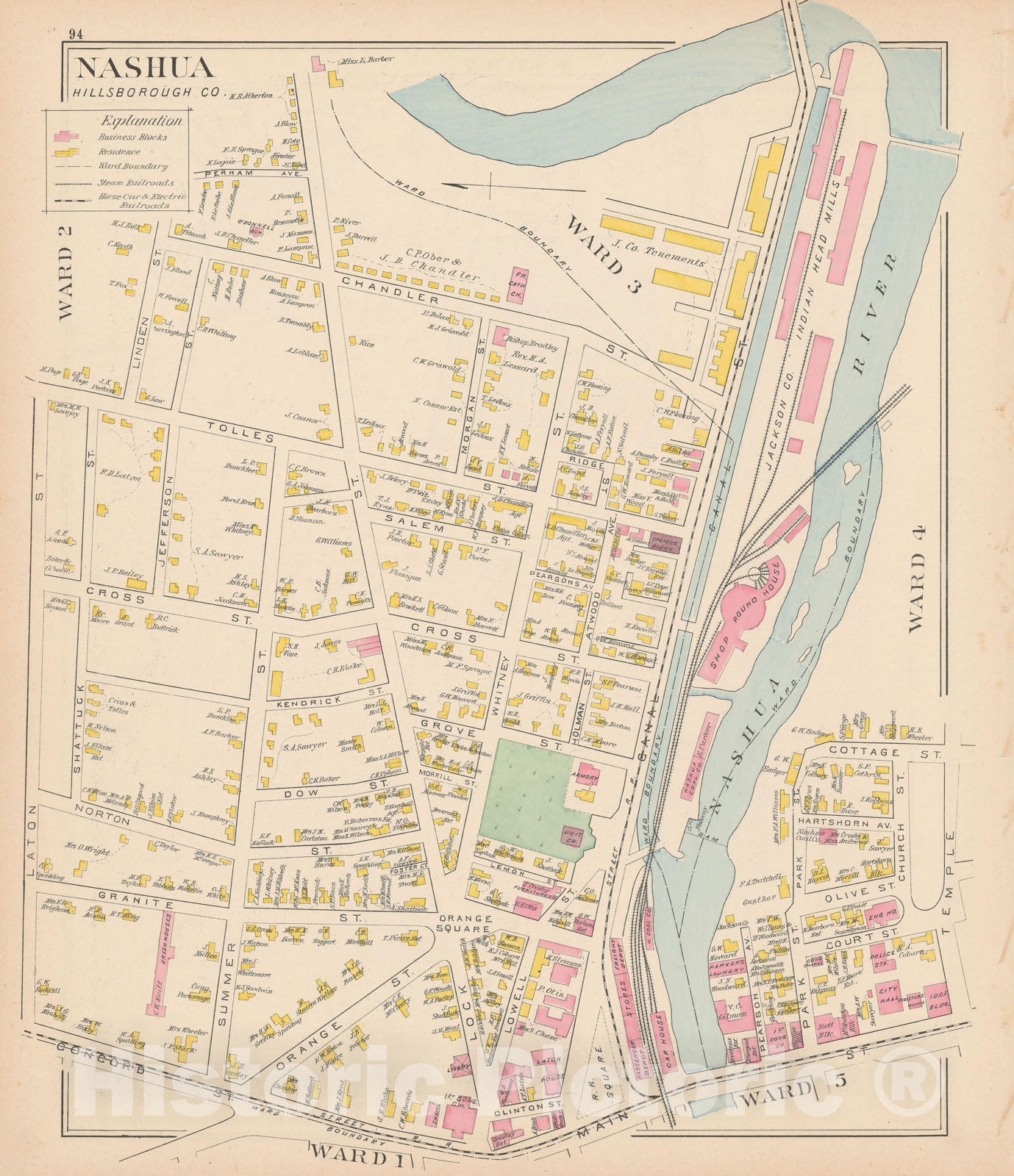This detailed antique map of Nashua in Hillsborough County is rendered on an old, tan, beige background with a dual-layered black border and a “94” inscribed at the top. The title "Nashua Hillsborough Co." is prominently displayed below the border. The map is sectioned into five wards: Ward 1 at the bottom, Ward 5 at the bottom right, Ward 4 in the middle right, Ward 3 in the center-top, and Ward 2 in the upper left. The Nashua River, marked with flowing white cloud-like graphics, cuts through the map from the bottom, curving up along the right-hand side and veering slightly left at the top.

The map's key at the top indicates that pink buildings represent businesses, while yellow ones denote residential structures. Streets like Chandler, Tolles, Salem, Cross, Grove, Kendrick, Dow, and Norton snake through the wards, with notable anomalies like the angular roads creating triangular sections. An orange square towards the bottom, alongside other labeled streets such as Cottage, Temple, Olive, and Court, punctuates the layout.

Buildings and residences are vividly contrasted in dark pink and yellow pastels, making this map stand out with an unusual yet detailed aesthetic. Additionally, a watermark at the bottom reads "Historic Pictoric®," ensuring the historical authenticity and vintage charm of the map.